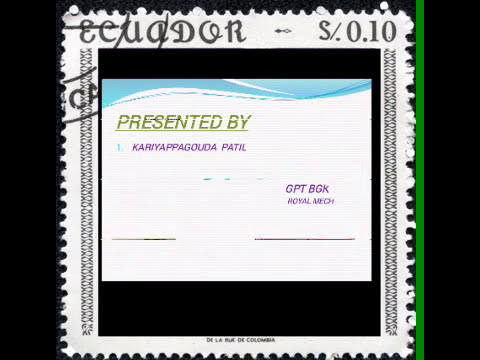The image depicts a stamp set against a black background, characterized by its jagged, perforated edges reminiscent of traditional postage stamps. The stamp features a prominent white border, with a thin vertical green stripe along its right edge. At the top of the stamp, "Ecuador - S. 0.10" is printed in black font. The left border of the stamp contains the letters "CA." Inside the stamp, decorative elements such as 'X's and small ornate details frame the main content. Two horizontal black stripes traverse the stamp's upper and lower sections. A larger gold text reads "Presented by," followed by the name "Caria Pagoda Patil" in purple font beneath it. At the bottom, in green font, it states "GPT BGK Royal Mech." The stamp’s intricate design includes a small swirl resembling an ocean wave near the top, adding to its decorative appeal.